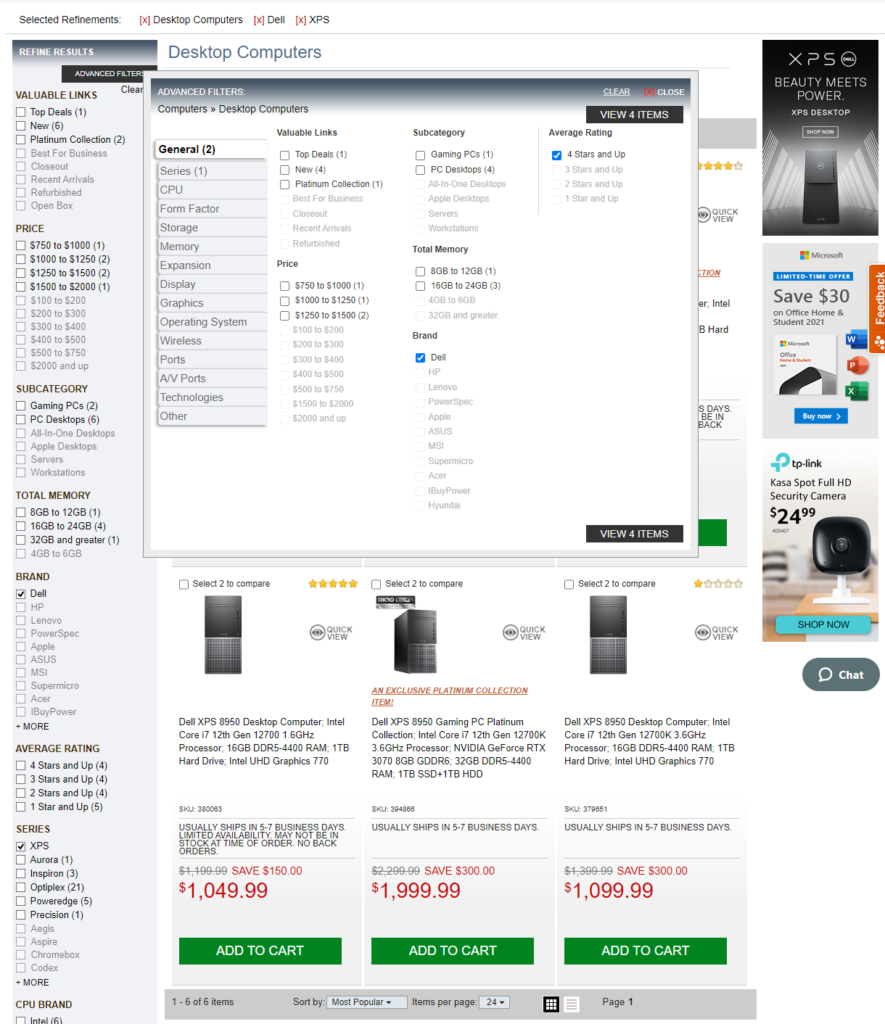In the screenshot, we observe a comprehensive interface for shopping for desktop computers and electronics. Beginning at the upper left, there are advanced filtering options including 'Valuable Links,' 'Top Deals,' and 'New Platinum Collection.' Below these, several price categories are listed: $750 to $1,000 with one item, $1,000 to $1,250 with two items, $1,250 to $1,500 with two items, and $1,500 to $2,000 with one item. 

Further down, there are subcategories like 'Gaming PCs,' which has two items, and 'PC Desktops,' featuring six options. Additional filters include 'Total Memory,' 'Brand,' and 'Average Ratings.' Under the 'Brand' filter, 'Dell' is selected, indicated by a checkmark next to its name. For the 'Series' filter, the 'XPS' series is selected, also marked with a checkmark. Lastly, the 'CPU Brand' category is listed at the bottom, ready for user selection.